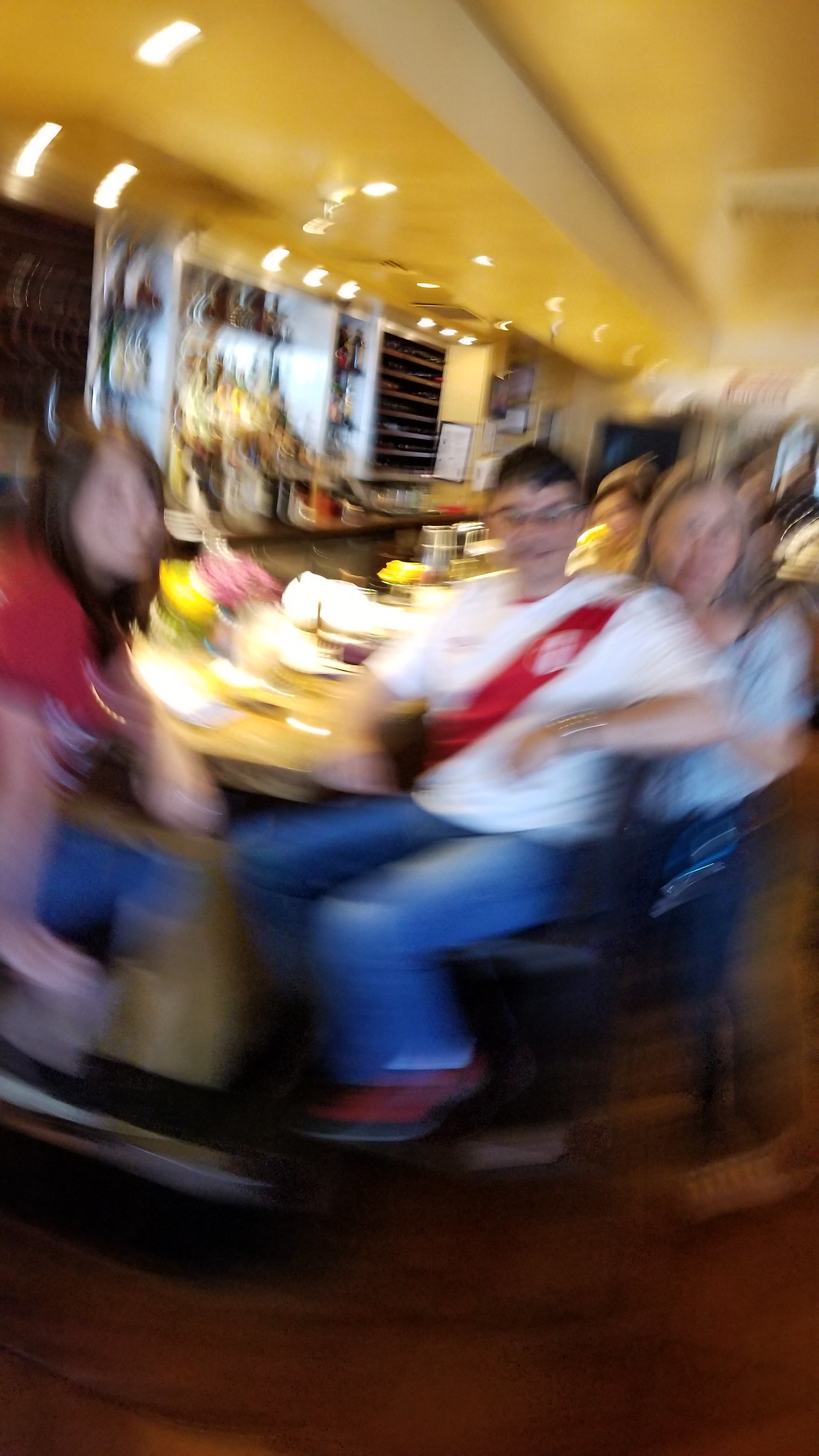This blurry and distorted photograph captures a lively scene of friends seated at a long dining table, possibly at a restaurant or in a house. The image is vertically oriented and features a unique blur effect that makes it appear as though the scene is spinning. Overhead, yellow downlights run along the ceiling, contributing to the warm ambiance. 

At the forefront to the left, a woman with long brown hair, wearing a red t-shirt and blue jeans, smiles directly at the camera. To her right, a young man with short black hair, glasses, and a white t-shirt with a red diagonal stripe (resembling a football jersey), also smiles while wearing blue jeans and red sneakers. To the right of him, a woman with straight blonde hair is seen in a short-sleeved, light blue top and dark brown trousers. The table they are seated at is cluttered with indistinct food items, glassware, and flowers, suggesting a social gathering or celebration. 

In the background, more blurry figures can be seen, adding to the sense of a crowded, convivial setting. Against the left wall, a bar area is partially visible, featuring shelves with bottles and perhaps shells, though details are obscured by the blur. The overall effect of the blur creates a kind of concentric ring pattern that distorts the edges and adds a dynamic, almost whimsical quality to the photograph.